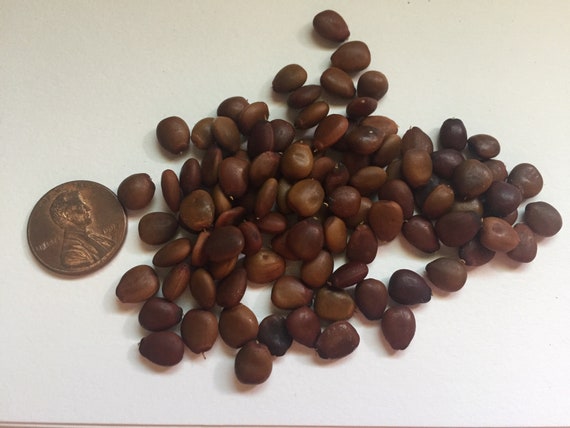The image depicts a collection of bulbous objects, suspected to be engorged ticks due to their circular, squishy appearance and small, leg-like appendages emerging from the front. They are grouped together on an off-white, heavy cardstock surface. To the left of the scene, a copper penny from the 1990s, with Lincoln’s profile visible, offers a size comparison, revealing that these objects are about one-fourth the size of the penny. The objects are clustered together, and despite their resemblance to rocks or beans, the presence of legs suggests they are indeed ticks. The lighting in the image casts shadows to the lower left, further emphasizing the rounded, almost polished surfaces of the ticks. The bottom of the image is partly clipped, showing the edge of the cardstock.